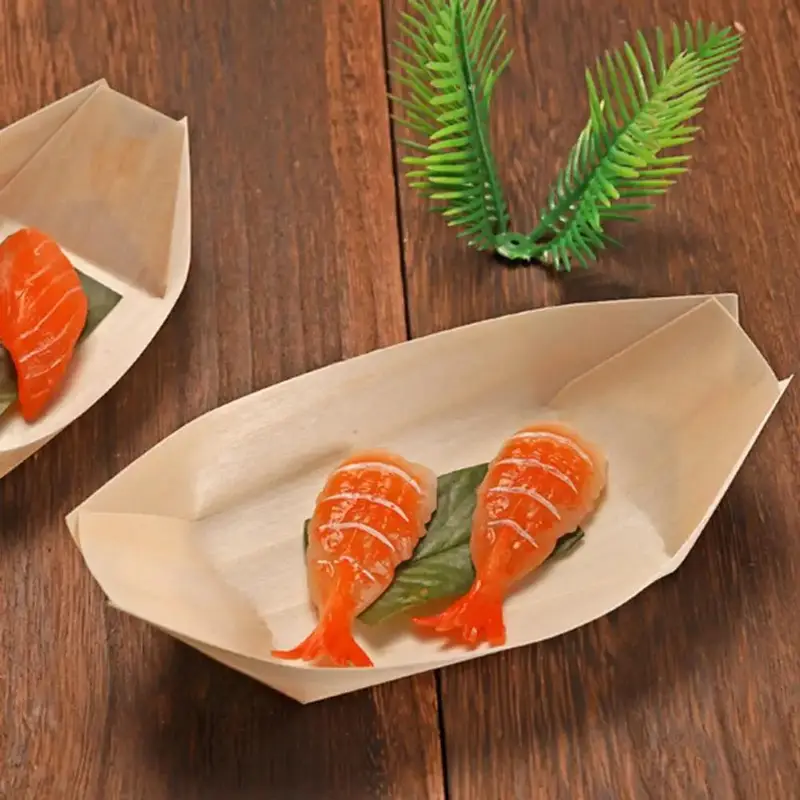The image showcases a pair of plates positioned on a dark brown, wood-like surface. Dominating the center of the photograph is a white, boat-shaped container. Inside this container lies a green leaf, upon which rests two pieces of orange, moist sushi that resemble the back halves of fish, complete with tails and white stripes. To the top right, a piece of decorative green plastic, appearing like fake pine needles, adds a touch of faux greenery. Just visible in the top left corner is a partial view of another white container, also lined with a green leaf and holding what appears to be a small piece of red, raw fish.